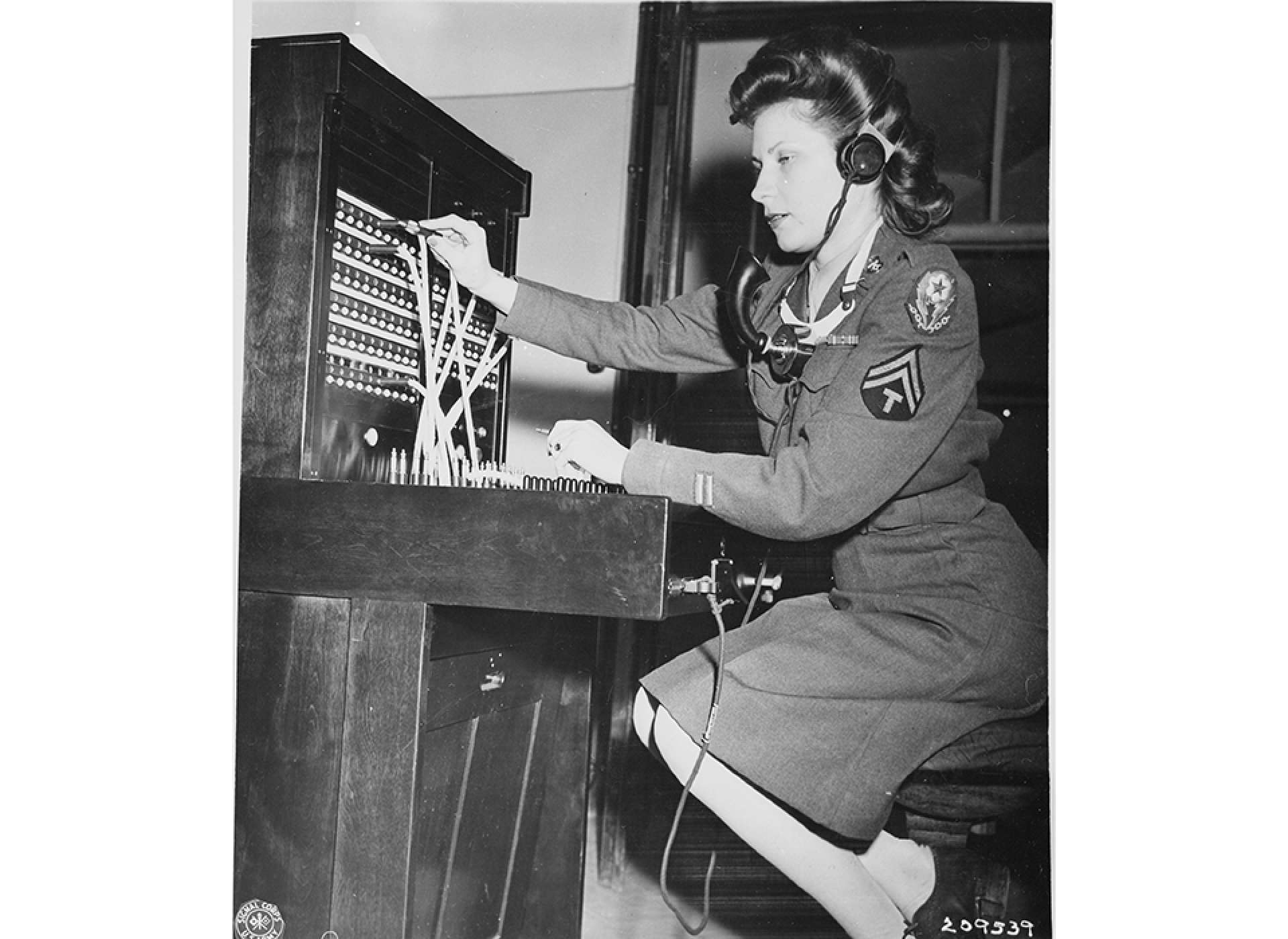The black and white photograph depicts a woman from the World War II era, working at an old-fashioned switchboard. She is seated, facing to the left, with her right arm engaged with the switchboard plugs and her left arm resting on the table. She wears a service uniform, possibly military, as indicated by the patches on her left arm and the coat adorned with military symbols. She also has a headset with a microphone on, suggesting she is managing communications.

The switchboard is large, taking up much of the left side of the image, with various wires and plugs extending towards the woman's midsection. Behind her is what appears to be a window with dark trim, through which nothing is visible outside. There is also a cabinet or shelving unit in the background. In the bottom right corner, the numbers "209539" are inscribed. Her medium-length brown hair is styled in a fashion typical of the 1930s or 1940s, adding to the historical ambiance of the scene. The overall setting suggests she is possibly operating the switchboard for the military, facilitating communication during the war.